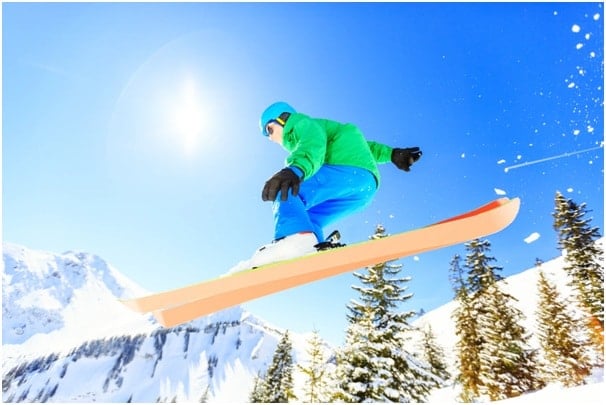The image captures an exhilarating moment outdoors on a ski slope, showcasing a skier mid-jump, performing a trick. The point of view is from the ground looking up, highlighting the skier in a dynamic pose with orange skis and a full winter outfit, including a green jacket, blue helmet, blue pants, and black gloves. The skier is positioned directly in the center of the image, slightly angled sideways, with pieces of snow trailing off the back of their skis. The scene is filled with vibrant colors, including different shades of blue, green, yellow, white, gray, brown, and a touch of orange.

In the background, the bottom left of the image features distant, snow-covered mountains, while the bottom right is adorned with several tall, green pine trees dusted with snow. The top part of the image showcases a clear, blue sky with a hazy sun positioned to the left of the skier's head. There is no text on the image, allowing the vivid and action-packed scene to fully captivate the viewer.